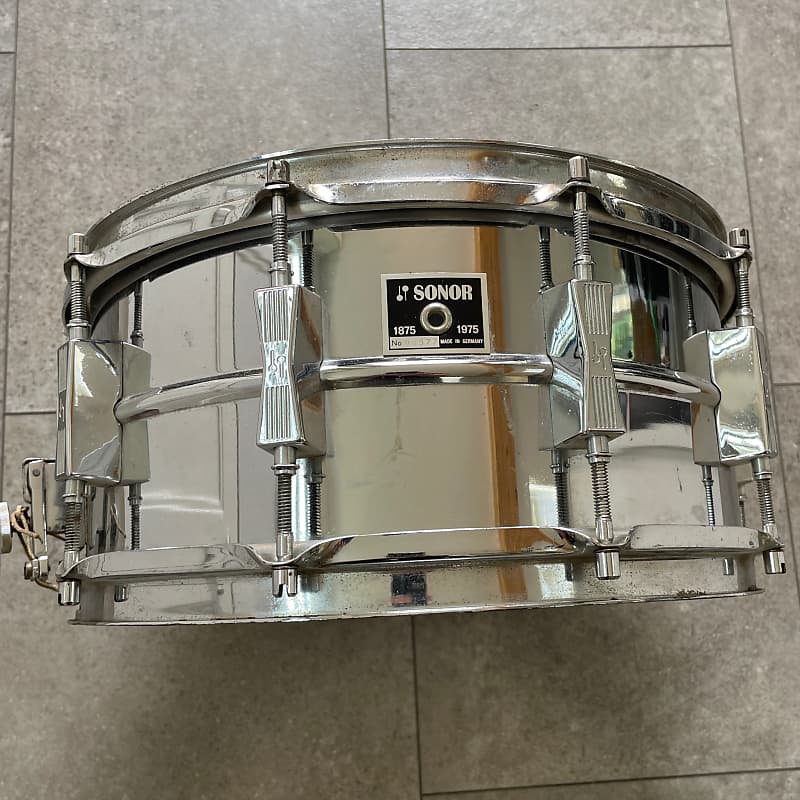This image showcases a close-up view of a shiny, stainless steel snare drum positioned on its side on a large, gray, square-tiled floor. The reflective surface of the drum captures the surrounding environment, hinting at a nearby wall and possibly a doorway. The drum features prominent screws running vertically from its bottom to top, with at least four visible. A clip on the left side of the drum appears to help secure its material. Centrally located on the drum's surface is a black label featuring the silver text "Sonor," flanked by the years "1875" on the left and "1975" on the right. Beneath the label's central black circle, there is a faintly imprinted silver triangle with numbering too small and faint to read clearly. To the right, the label indicates "Made in," although the country of origin remains indistinguishable due to the small print. Parts of the drum gleam under the light, enhancing its metallic luster.